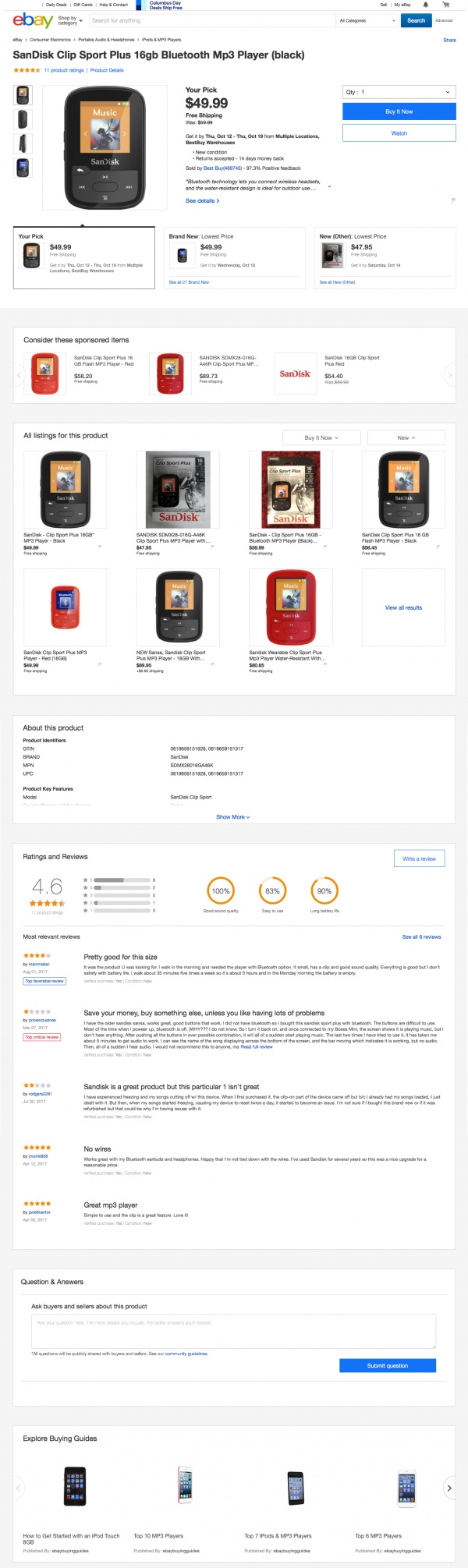Screenshot of an eBay product listing for a SanDisk Clip Sport Plus 16 GB Bluetooth MP3 Player in black. The listing prominently displays "Your Pick" alongside a price of $49.99 with free shipping. The estimated delivery window is from Thursday, October 12th to Thursday, October 19th, and the item is available from multiple locations. On the left side of the screen, there are four thumbnail images of the MP3 player from different angles, with the top image selected, showing the player displaying a music screen and the SanDisk logo. The interface includes interactive elements such as a quantity selector set to one, a blue "Buy It Now" button, and a white "Watch" button.

Further down the page, there's a section labeled "All Listings," showcasing related sponsored items. User reviews are highlighted, with the product boasting an average rating of 4.6 stars. The reviews are available for reading. At the bottom, there's a Q&A section where users can submit their questions via a blue "Submit Question" button.